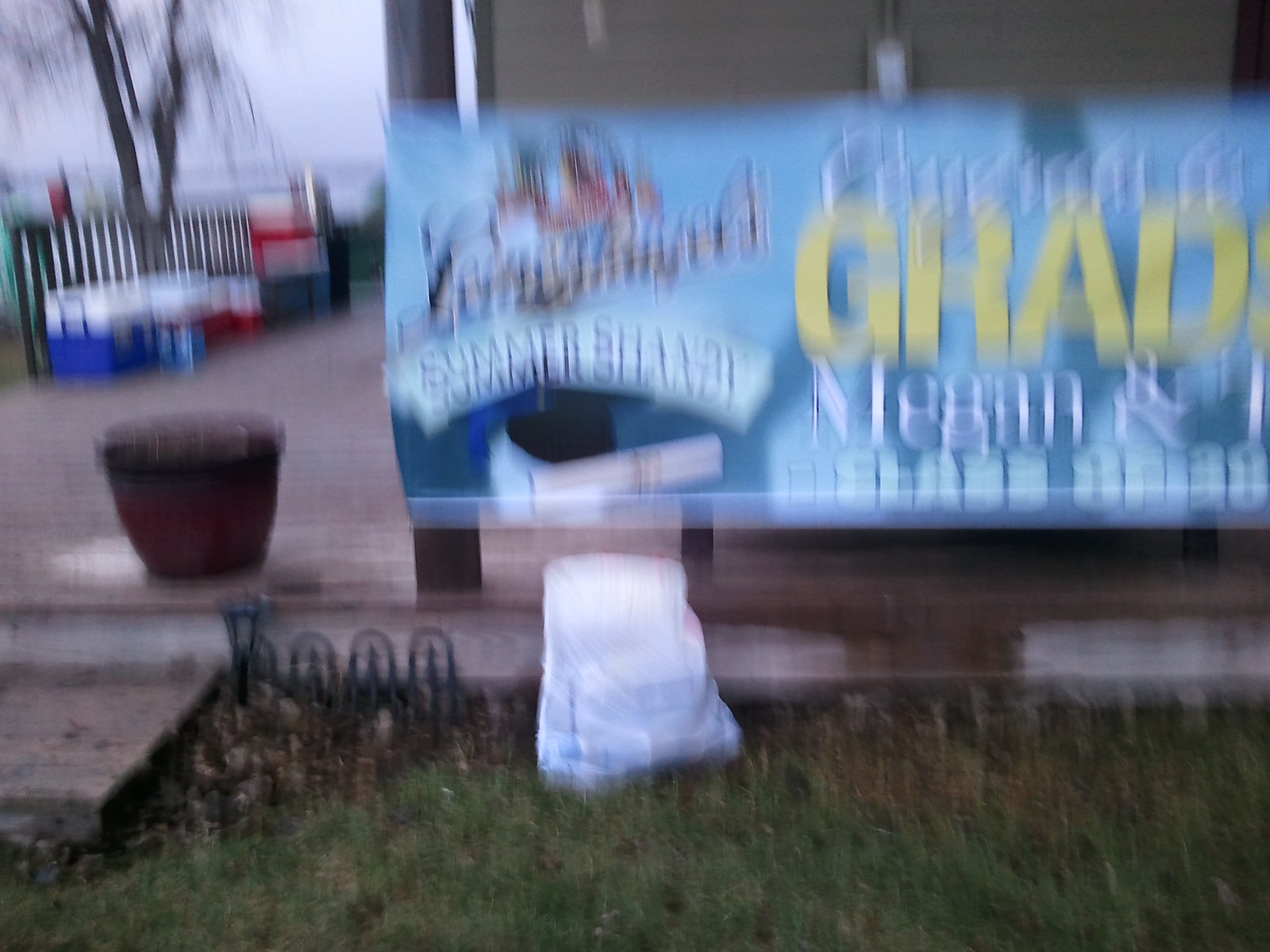The photograph, taken outdoors, depicts a small, billboard-like sign attached to a tan-sided building with dark wooden edges. The sign features a blue patterned background with capital yellow letters spelling "GRAD." Above it, the word "CONGRATULATIONS" is visible, and below it, the name "MEGAN" can be discerned despite the blurriness. Additional blurry text includes phrases like "SUMMER," "SHANDY," and "SUMMER SHANDY." The sign is supported by dark wooden posts and stands next to a brown planter on the left, with a white plastic bag and some coolers (one blue, one red) on the ground nearby. To the right, there’s a deck or porch with steps leading up, and below it, unkempt grass and weeds. In the background, a v-shaped tree hints at a beachfront location, with clear blue sky visible in the top left corner.